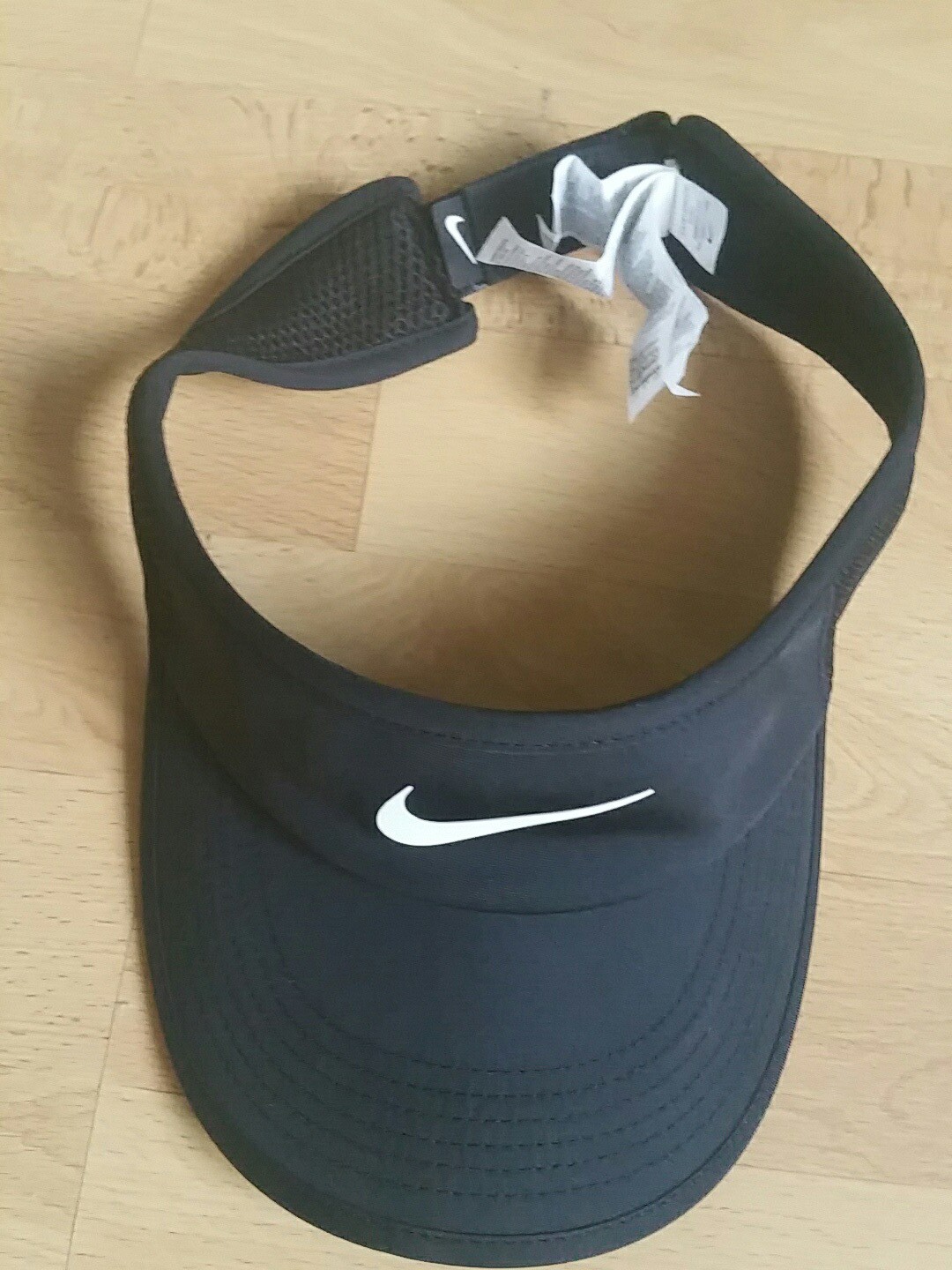This photograph captures a close-up view of a black Nike visor, commonly worn for sports like tennis or golf. The image is taken from above, highlighting the top and front of the visor which prominently features a white Nike swoosh centered above the bill. The visor, designed with a narrow strip that goes around the head and adjustable fastening at the back, rests on a butcher block style surface. The surface, either a tabletop or floor, has a pale pine-like color, constructed with rectangular sections in an inlaid pattern. Visible on the inner part of the visor are several long white tags with small black print, likely containing washing and material information. The scene is well-lit, casting subtle shadows from the visor onto the light wooden surface, suggesting a bright light source in the room.